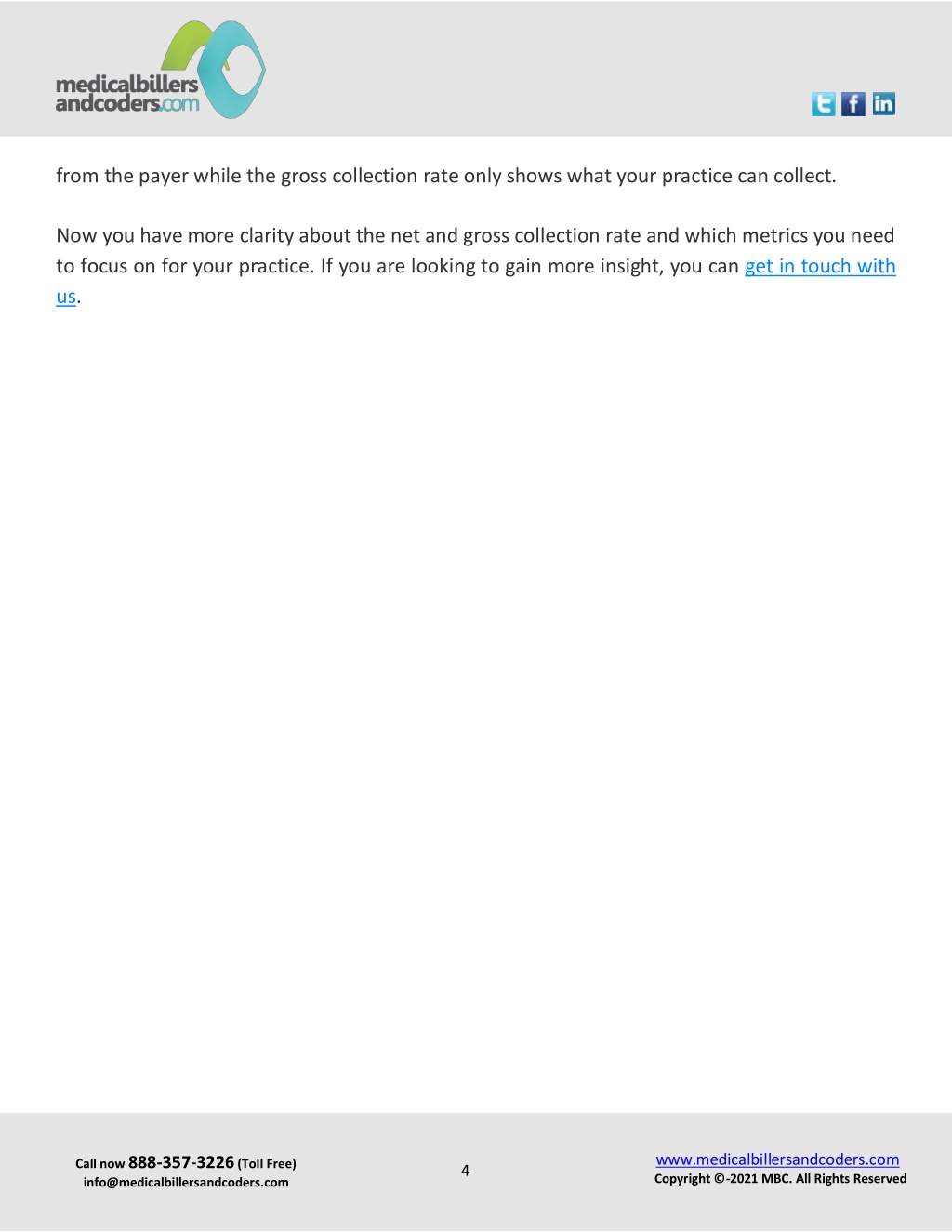In the image, a grey box is situated at the top, featuring the text "medicalbillersandcoders.com" in black font on the left side. The ".com" portion of the URL is highlighted in blue. Above this text, there is a green semi-circle, and adjacent to it, a uniquely shaped blue circle with a powder blue outer ring and a greyish background inside. To the right of these elements are the logos for Twitter, Facebook, and Indeed.

Beneath this, in small black font, the text reads: "From the payer, while the gross collection rate only shows what your practice can collect." On the next line, it continues: "Now you have more clarity about the net and gross collection rate and which metrics you need to focus on for your practice. If you are looking to gain more insight, you can." The phrase "get in touch with us" is underlined in blue.

A white background spacer extends from here down to the next grey box. On the left side of this box, small black font reads: "Call now 888-357-3226 (toll-free)." Below this, it says "info@medicalcalibersandcoders.com." Further to the right, the number "4" appears, and to the right side again, it reads "www.medicalbillsandcoders.com" in blue underline. Underneath this, the text in black font states: "© 2021 MBC. All Rights Reserved."